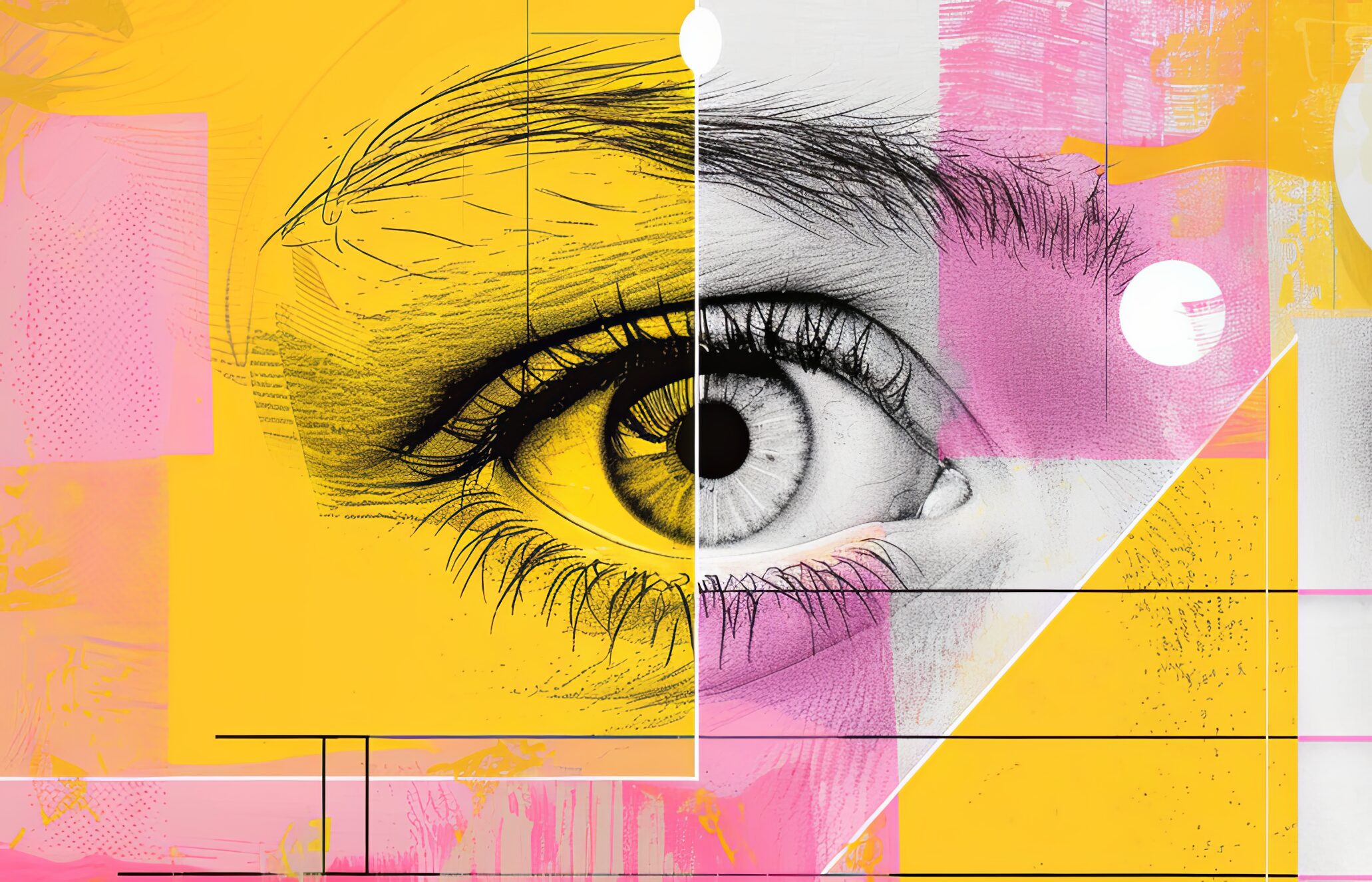This artwork features a highly detailed, realistic pencil drawing of a human eye at its center. The eye, which appears to belong to a person with light-colored, possibly blue, eyes, includes meticulously drawn individual hairs in the eyelashes and a structured iris. The black and white eyebrow above the eye displays slight wrinkles and stray hairs that suggest natural growth. Superimposed over this monochrome depiction are transparent geometric shapes and colorful elements. A yellow square partially covers the eye, while a yellow triangle is situated near the right corner of the image. At the top right-hand side, a pink rectangle adds to the vibrant overlay. Various shapes, including an orange triangle and irregular forms, along with several black lines and a single white line featuring an oval, crisscross the artwork. The background also contains a bright, moon-like illuminated circle, enhancing the composite, multimedia nature of the piece with its juxtaposition of pencil sketch realism and digitally painted, mod-like geometric abstractions.